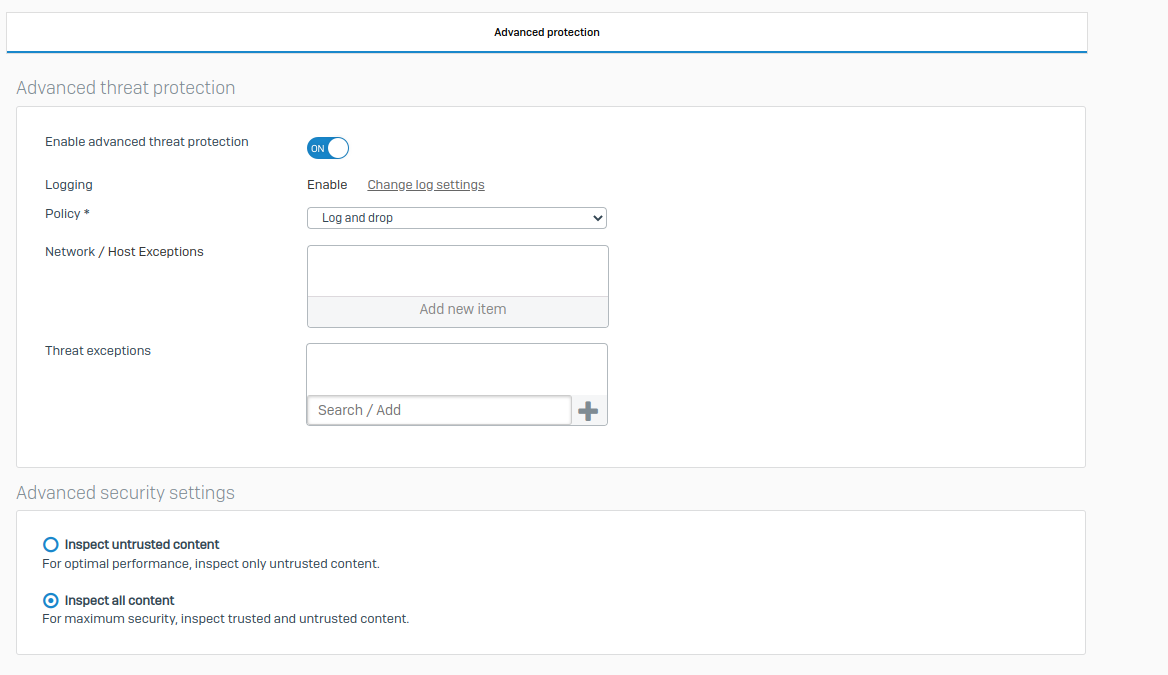This screenshot captures the interface of an unidentified website focused on advanced security settings. At the top of the interface, the heading "Advanced Protection" is prominently displayed. Below this heading, a thin blue horizontal line spans the entire width of the image.

On the left side, various security options and configurations are listed in detail:

1. **Enable Threat Protection and Enable Advanced Threat Protection**: These settings are currently activated, as indicated by the slider button being in the "On" position.

2. **Logging**: Options provided are to enable logging and change log settings.

3. **Policy Settings**: The current policy is set to "Log and Drop".

4. **Network/Host Exceptions**: Users can add new items to this list.

5. **Threat Exceptions**: Users have the ability to search or add new items here.

Under the section labeled "Advanced Security Settings", there are two configurations for content inspection:

1. **Inspect Untrusted Content**: This option is chosen to ensure optimal performance by inspecting only untrusted content.
   
2. **Inspect All Content**: This setting, which is not selected, would offer maximum security by inspecting both trusted and untrusted content.

Notably, the image lacks any photographic elements and follows a minimalist design focused solely on text and interface components. The dimensions of the screenshot suggest that it is wider than it is tall. The image contains no human, animal, bird, plant, or automotive elements.